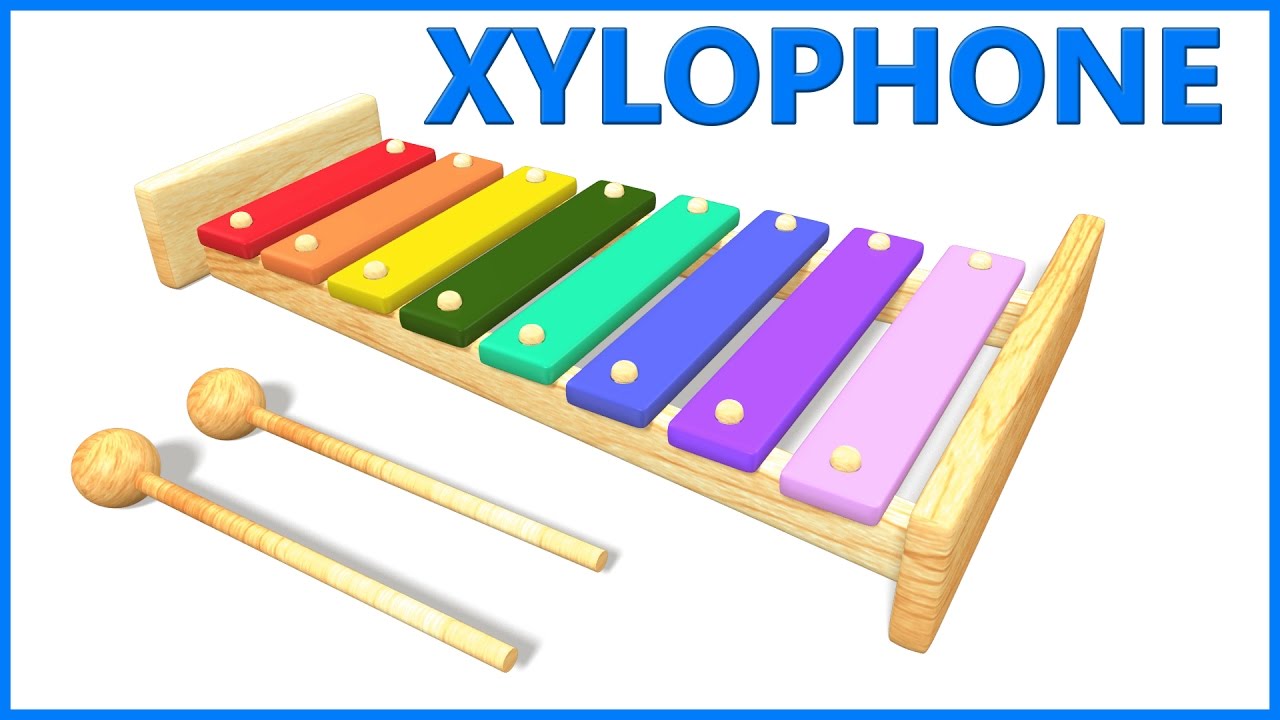This is a professionally created drawing of a xylophone labeled in bold blue letters "XYLOPHONE" at the top right. The illustration showcases the instrument set against a plain white background, providing no context for its setting. The xylophone itself features a wooden frame with eight keys of varying colors, arranged from left to right in an ascending size from small to large. The keys progress through a spectrum of colors: red, orange, yellow, dark green, light green, turquoise, blue, purple, light lavender, and pink. Below the keys, positioned in front of the xylophone, are two light wooden mallets used to strike the keys to create sound. Encompassing the whole image is a thin blue border.